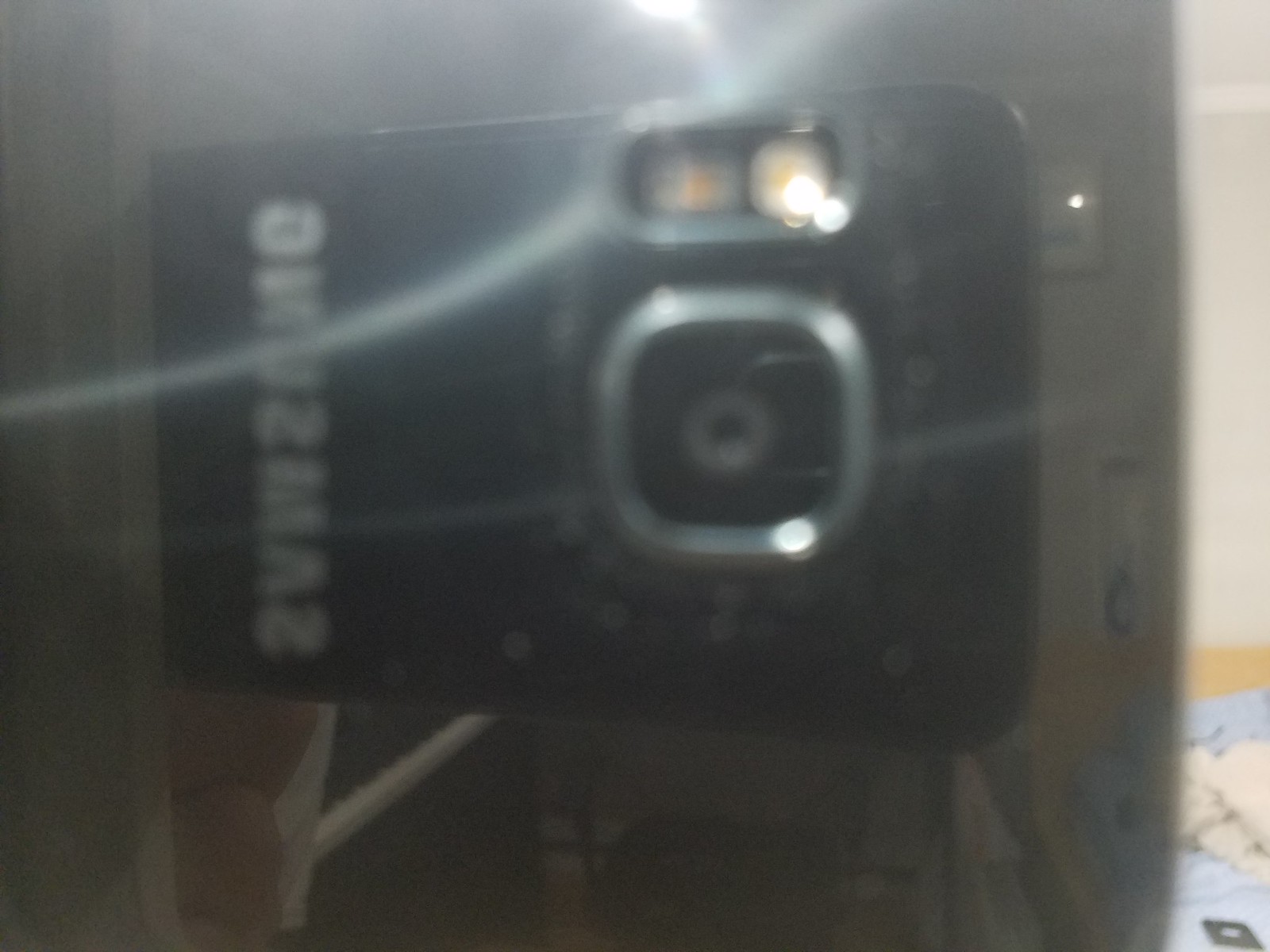This photograph depicts a blurry and washed-out image, likely taken in a bedroom, featuring a Samsung phone. The phone, characterized by its dark gray, glossy exterior, is distinguished by the prominent Samsung logo, which appears in lighter gray text. The main camera on the phone boasts a large lens encircled by a silver rim, accompanied by a flash. The blur and distortion of the image suggest it might have been captured through a reflective surface, possibly a mirror or window, resulting in noticeable light rays emanating from a light source, likely a room fixture.

In the background, the setting appears to be a bedroom, discernible by the white-painted walls adorned with posters and a bed situated to the right. The bed features a wooden frame in a lighter brown hue, topped with blue or blue-striped bedding, and a couple of white pillows. The lower right corner of the image hints at the presence of another device, perhaps another cell phone or tablet. Despite the indistinctness of the photo, subtle details, such as a slight reflection of the person holding the phone, can be made out.